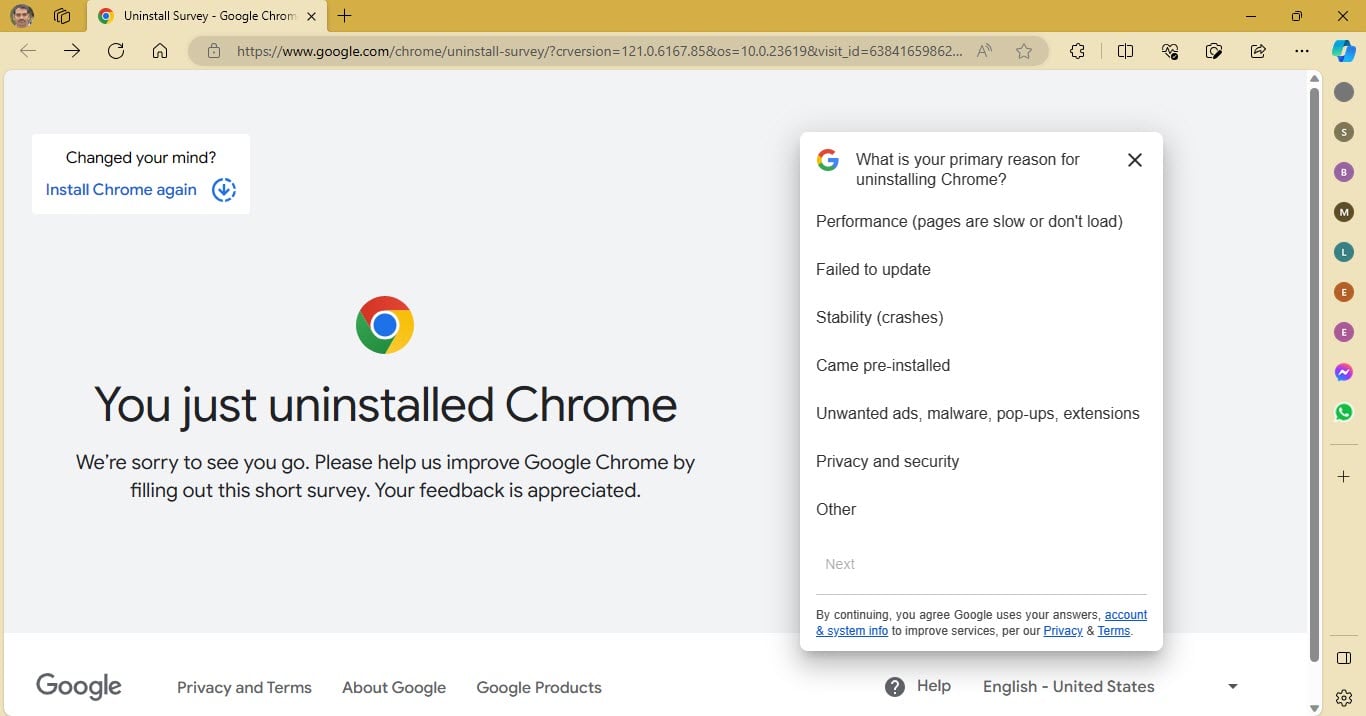The website displayed is Google Chrome's uninstall survey, accessible at [googlechrome.com/chrome/uninstall-survey](https://googlechrome.com/chrome/uninstall-survey). The top left corner features a message "Changed your mind?" accompanied by a button prompting users to "Install Chrome again."

The browser being used appears to be a Microsoft browser, likely Microsoft Edge, although this is not certain. The main content of the page indicates that the user has just uninstalled Chrome, stating, "We're sorry to see you go. Please help us improve Google Chrome by filling out this short survey. Your feedback is appreciated."

To the right, there is a small survey box. At the top of the survey, it asks "What is your primary reason for uninstalling Chrome?" followed by multiple choice options including:
- Performance: Pages are slow or don’t load
- Failed to update
- Stability: Crashes
- Came preinstalled
- Unwanted ads
- Malware: Popup extensions
- Privacy and security
- Other

Below the survey, privacy policy text is visible. The bottom bar of the page displays a grayscale Google logo, links for Privacy and Terms, About Google, Google Products, and a help button. Additionally, there is a language switcher currently set to "English (United States)."

Uniquely, the taskbar of this computer is positioned on the right side of the screen, rather than at the bottom as is more common.